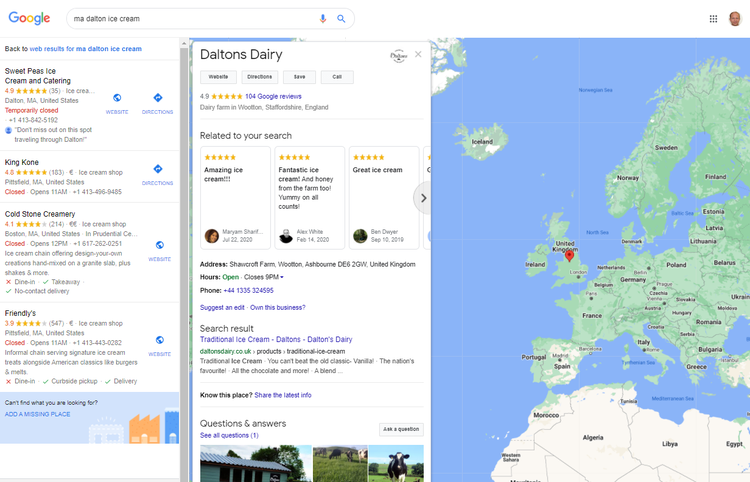Sure, here's a detailed and cleaned-up caption for the image:

---

The image displays a Google search results page on a computer screen. In the upper left corner, the recognizable colorful Google logo is visible. Below the search bar, the user has searched for "Ma Dalton Ice Cream," leading to a series of results about ice cream shops and related businesses.

On the left side of the page, there are several search results listings for various ice cream establishments:

- **Sweet Peas Ice Cream and Catering**, located in Dalton, Massachusetts
- **King Cone**, based in Pittsfield, Massachusetts
- **Cone Stone Creamery**, situated in Boston, Massachusetts
- **Friendly's**, also in Pittsfield, Massachusetts

Each listing provides additional details about the respective establishments.

Dominating the right side of the screen is a prominent information panel about **Dalton's Dairy**. This panel indicates:
- **Dalton's Dairy** has a high rating of 4.9 stars.
- It includes various positive reviews with remarks such as "Amazing Ice Cream," "Fantastic Ice Cream," and "Great Ice Cream."
- The address is given as Shawcroft Farm, Wooten, Ashbourne, United Kingdom.
- It mentions that Dalton's Dairy is open until 9 PM.
- The panel includes a contact phone number.

Adjacent to this information panel is a map primarily depicting Europe, with portions of Africa visible. The United Kingdom, marked in green, features a red location pin indicating Dalton's Dairy's precise location.

---

This caption provides a detailed and structured description of the image, highlighting all relevant information visible on the Google search results page.